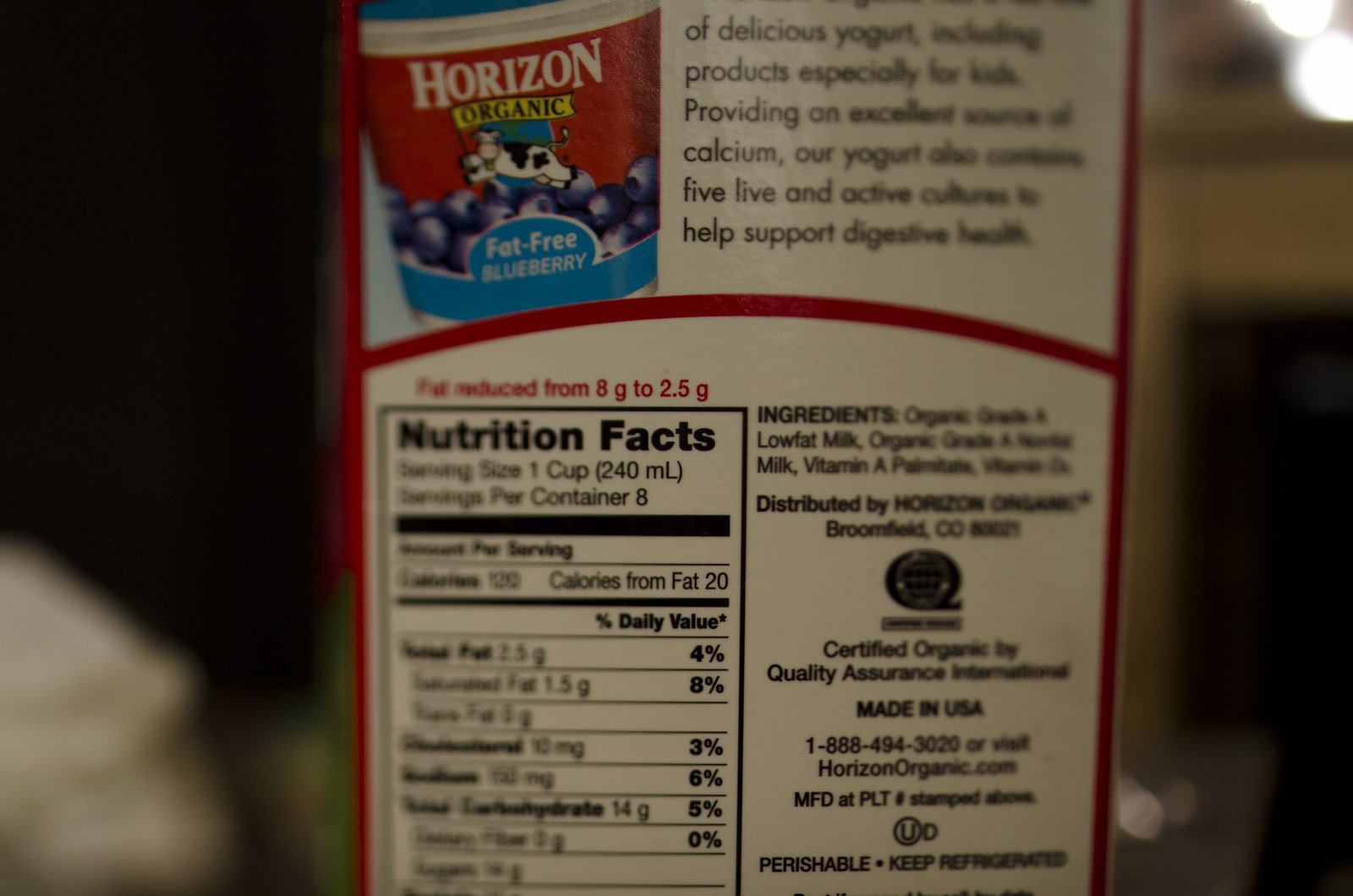This photograph features a close-up of the nutrition information for a product labeled "Horizon Organic Fat Free Blueberry Yogurt." The label highlights that this yogurt is specially formulated for kids and is touted as delicious while providing an excellent source of calcium. Additionally, the yogurt contains five live and active cultures to support digestive health. The ingredient list is included but not entirely legible due to some blurriness. 

On the left side of the label, the nutrition facts are also slightly blurry. However, it indicates that each serving is one cup (240 milliliters) and contains 120 calories, with 20 calories from fat. Notably, the text mentions that the fat content has been reduced from eight grams to two and a half grams. The product is made in the U.S., and consumers are advised to keep it refrigerated due to its perishable nature. The official website for the brand is horizonorganic.com, and the container includes a manufacturing stamp labeled "PLT." There is also a phone number provided for further inquiries.